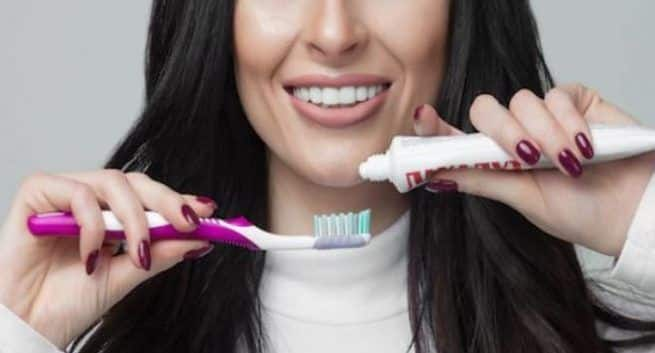A rectangular photo, horizontally aligned, showcases a smiling woman promoting dental hygiene. The top of the photo starts at the bridge of her nose and ends just above her chest, cutting off her eyes and focusing on her bright smile and white teeth. She has long, dark brown or black hair draping over her shoulders and wears a white turtleneck shirt with long sleeves. Her lips are pink and display an open mouth smile, highlighting her perfect white teeth. The woman's hands are raised to chin height, with all fingernails painted a dark burgundy or red color. In her right hand, she holds a pink and white toothbrush horizontally, its bristles white and blue. In her left hand, slightly higher, is a white uncapped tube of toothpaste, partially obscured by her thumb, clearly indicating she is about to apply the toothpaste to the toothbrush. The scene strongly suggests a promotion for brushing teeth to achieve a stunning, white smile like hers.